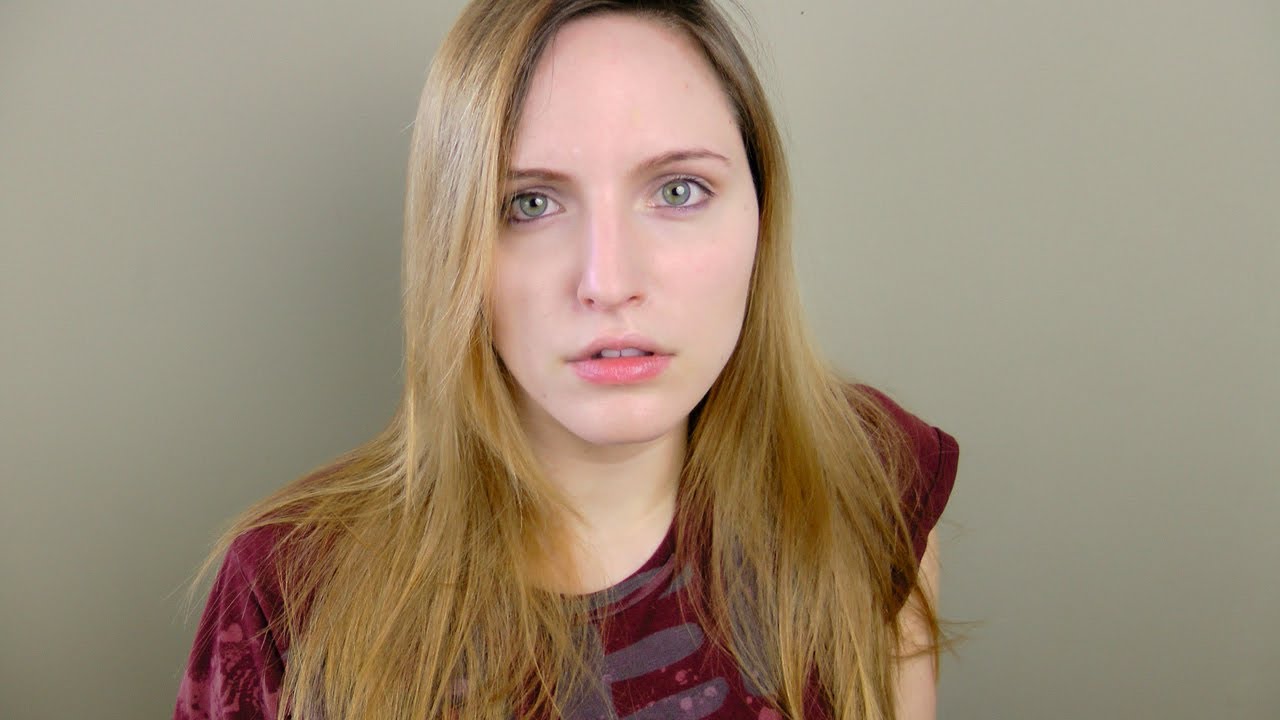The image depicts a woman with long, reddish-blonde hair that cascades down to her chest, wearing a distinctive purple corduroy-like shirt with a tie-dye effect featuring splashes of gray. She gazes directly into the camera, exuding a certain edge and intensity. Her light blue-gray eyes, highlighted with a hint of eyeshadow, convey an expression that seems to straddle between fear and an attempt to pose dramatically. Her lips, slightly parted and glossed, suggest a touch of effort in her presentation, though her overall makeup is minimal, lending her a more natural and raw appearance. The backdrop greets the viewer with a neutral beige-gray palette, further emphasizing the woman's striking presence and contrasting emotions.